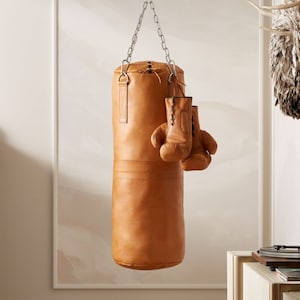This is a detailed photograph of a rustic room with off-white or ivory walls. In the center, a large, tan, brown leather punching bag hangs vertically from the ceiling, suspended by a sturdy silver chain. Attached to the chain on the right are a pair of matching brown leather boxing gloves, showcasing intricate stitches. To the right of the punching bag, there is a low wooden bench or chest with a white and brown finish, topped with a few thin books. Above it, affixed to the wall, is a feathery item, possibly a pelt or a scarf. In the bottom right corner of the image, a section of what might be a desk or table is visible, hinting at a cluster of objects neatly arranged on its surface. The room is softly lit, casting faint shadows that add depth to the corners. Overall, the setting appears clean and slightly rustic, blending an athletic focus with homely decor elements.